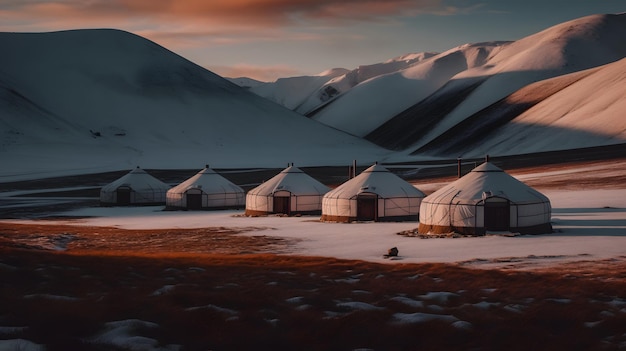This is an intricate painting depicting a barren, cold landscape consisting of five identical yurts or tents. The yurts are uniformly aligned, all facing towards the photographer. They are colored the same off-white as portions of the ground and feature a distinctive brown rim where the sides meet the tops. The terrain around the yurts is a stark contrast of deep brown and off-white, suggesting patches of snow dotting an orangish-red earth. In the background, there are barren hills or mountains, mostly covered in uniform white snow, with some brown areas peeking through. The sky showcases a striking feature—orange clouds in the upper left corner, adding a touch of warmth to this desolate, snowy scene. Overall, the image bears some evidence of being generated by AI, with its meticulous blending of colors and textures.